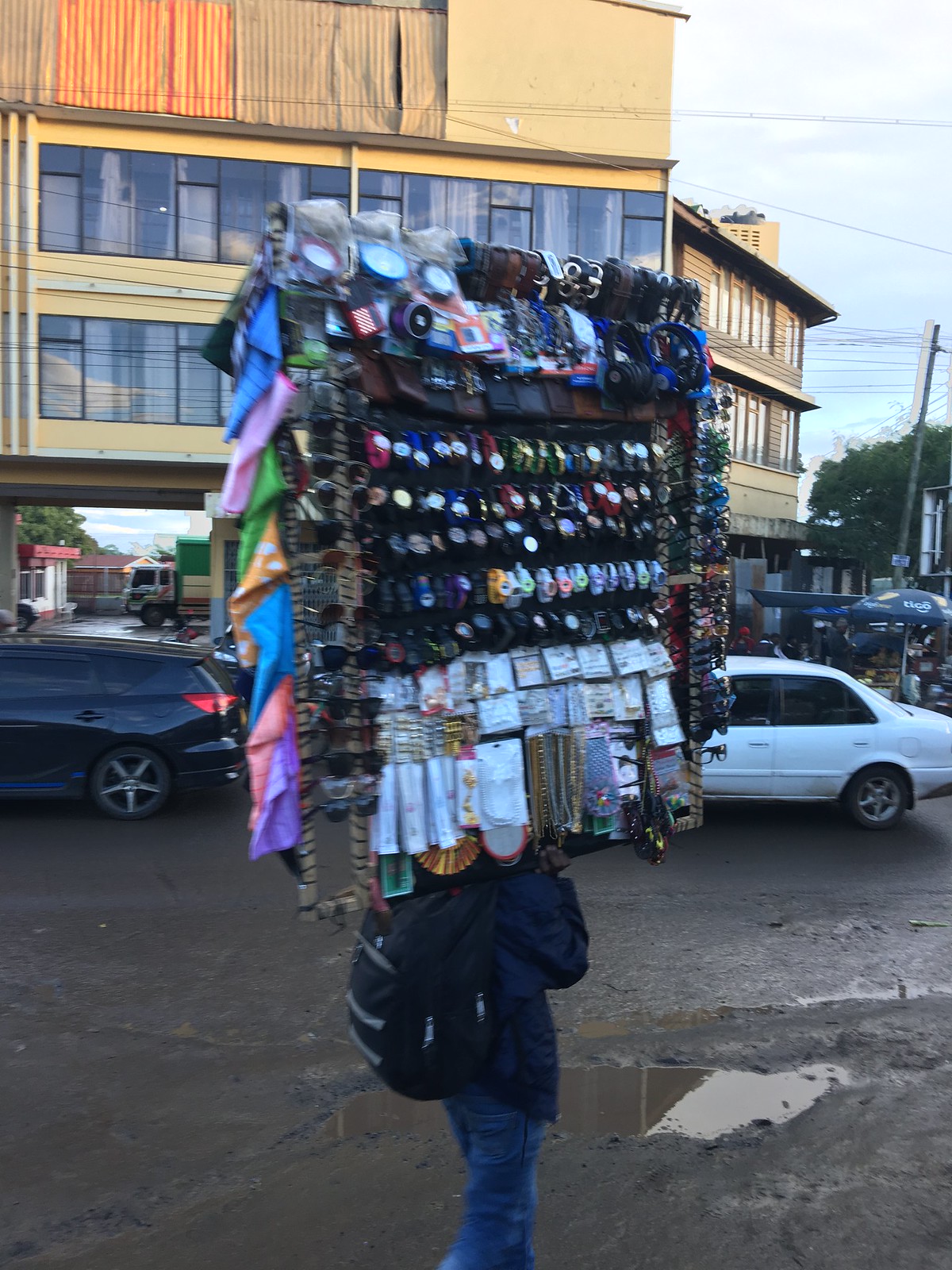In this image, a woman walks down a muddy, rain-soaked street, identified by a puddle in her path. She carries a large board on her head, laden with a variety of goods, suggesting she's an on-the-go vendor. The board holds an eclectic array of items: watches and glasses in the middle, handkerchiefs, scarves, and possibly hats and socks to the sides. She is dressed in a blue coat, blue jeans, and has a black backpack. In the background, a somewhat run-down, brownish yellow apartment building with drawn curtains stands behind two parked cars—a white one and a blue one. Additionally, a tree, an umbrella, and power lines punctuate the scene, adding details to this snapshot of daily life.